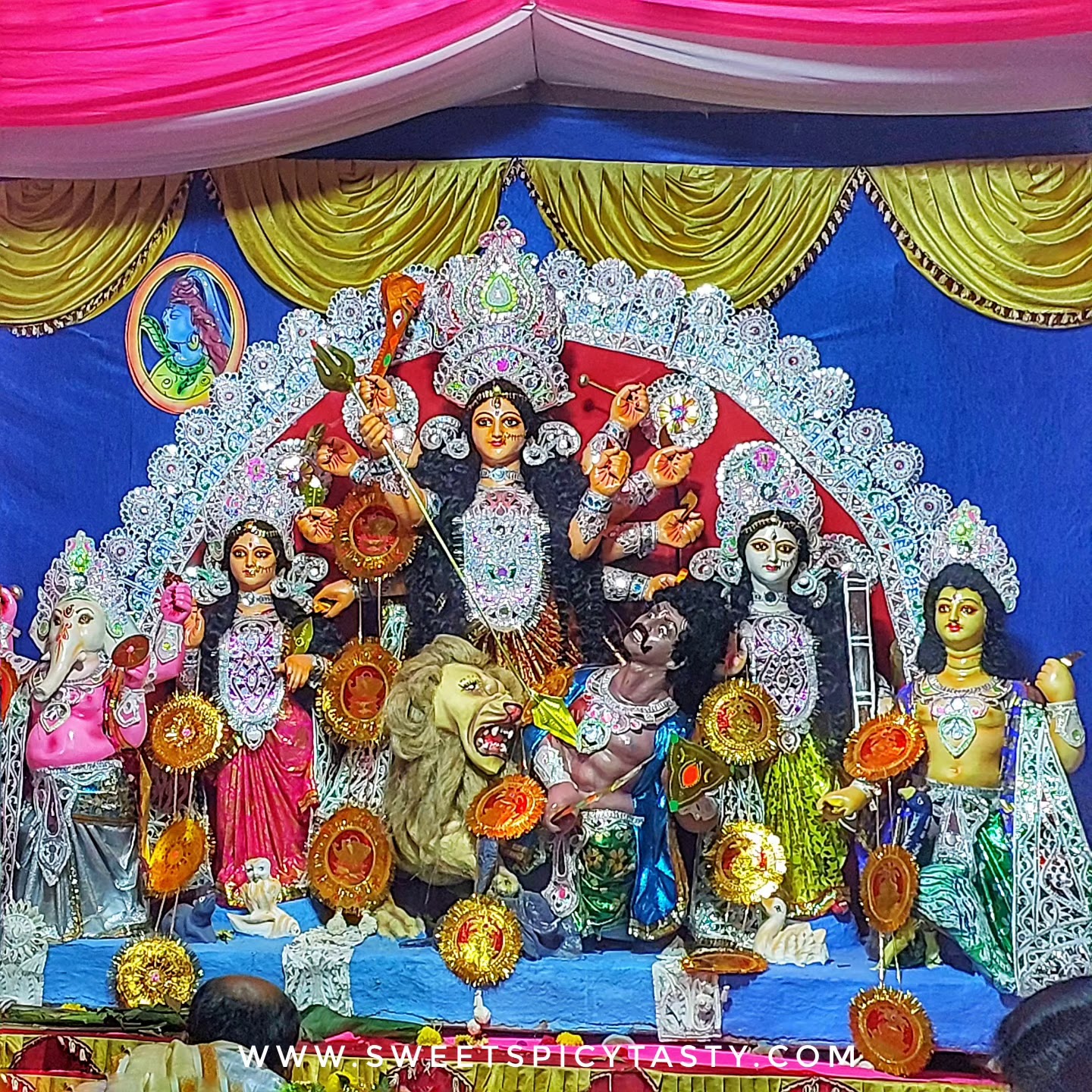This image depicts an elaborate, vibrant display likely set on the side of a circus wagon, showcasing a group of five intricately dressed mannequins resembling Indian figures. These figures, dressed in gaudy, traditional Indian garb adorned with sparkling, diamond-like baubles, stand in front of a semicircular backdrop. The mannequins include three women wearing glittery dresses in pink, blue, and green with white lace accents, all topped with lace headdresses. Two men, one of whom is a black man with a curled mustache and fuller hair, also don traditional outfits and dark makeup. The black man, appearing as a lion tamer, is depicted next to a fierce, growling golden lion, creating a dramatic scene of tension as if he is backing away in fear. Additionally, there is an elephant off to the side, completing the scene filled with vibrant colors and rich textures. The entire setting has a blue background embellished with draping gold banners, and at the bottom of the image, the website www.sweetspicytasty.com is prominently displayed. In front of the display, a few onlookers' heads can be seen, suggesting it is part of a public exhibition or performance, enhancing its dramatic and theatrical presentation.